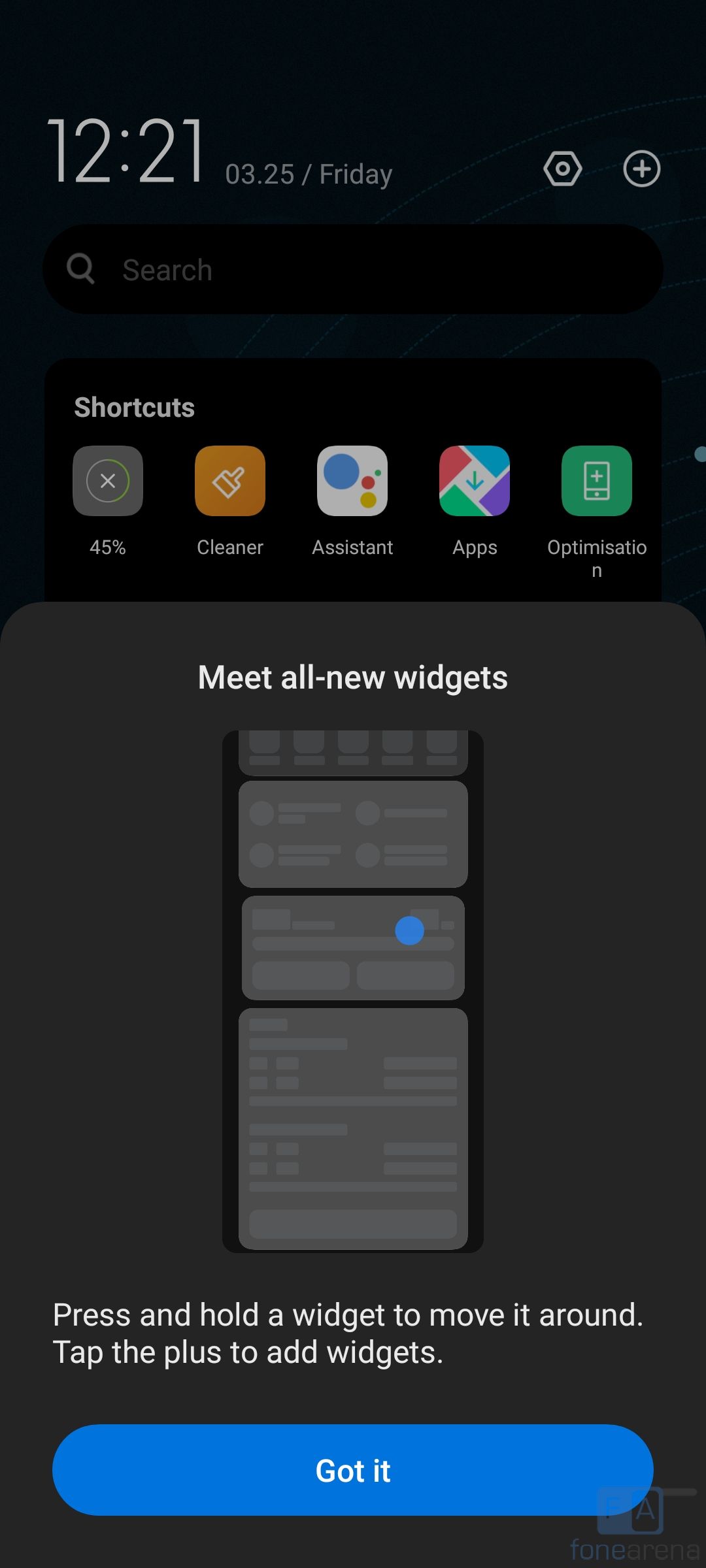The image showcases a vertical smartphone screenshot with various interface elements displayed. At the very top, the status bar features the time "12:21" in large white text, followed by the date "0325 / Friday." Flanking the top corners are two icons: a settings button on the left and a plus button on the right, both in white.

Beneath the status bar, a black search bar is prominently displayed, featuring the word "Search" in white text next to a light gray magnifying glass icon. Just below this, a row of app shortcuts appears against a darker background. The apps listed include "45% app," "Cleaner app," "Assistant app," "Apps app," and "Optimization app."

The lower half of the screen transitions to a dark gray background. Dominating this section is a "Meet All New Widgets" header in white text. Beneath this heading is a large, grayed-out silhouette icon of a phone screen. Further instructions are provided in white text: "Press and hold a widget to move it around. Tap the plus to add widgets."

Toward the bottom, the interface features a large blue button labeled "Got it," inviting user interaction. The entire screenshot is a tall rectangle with a length that extends vertically, with the dark gray section starting approximately at the midpoint of the image.